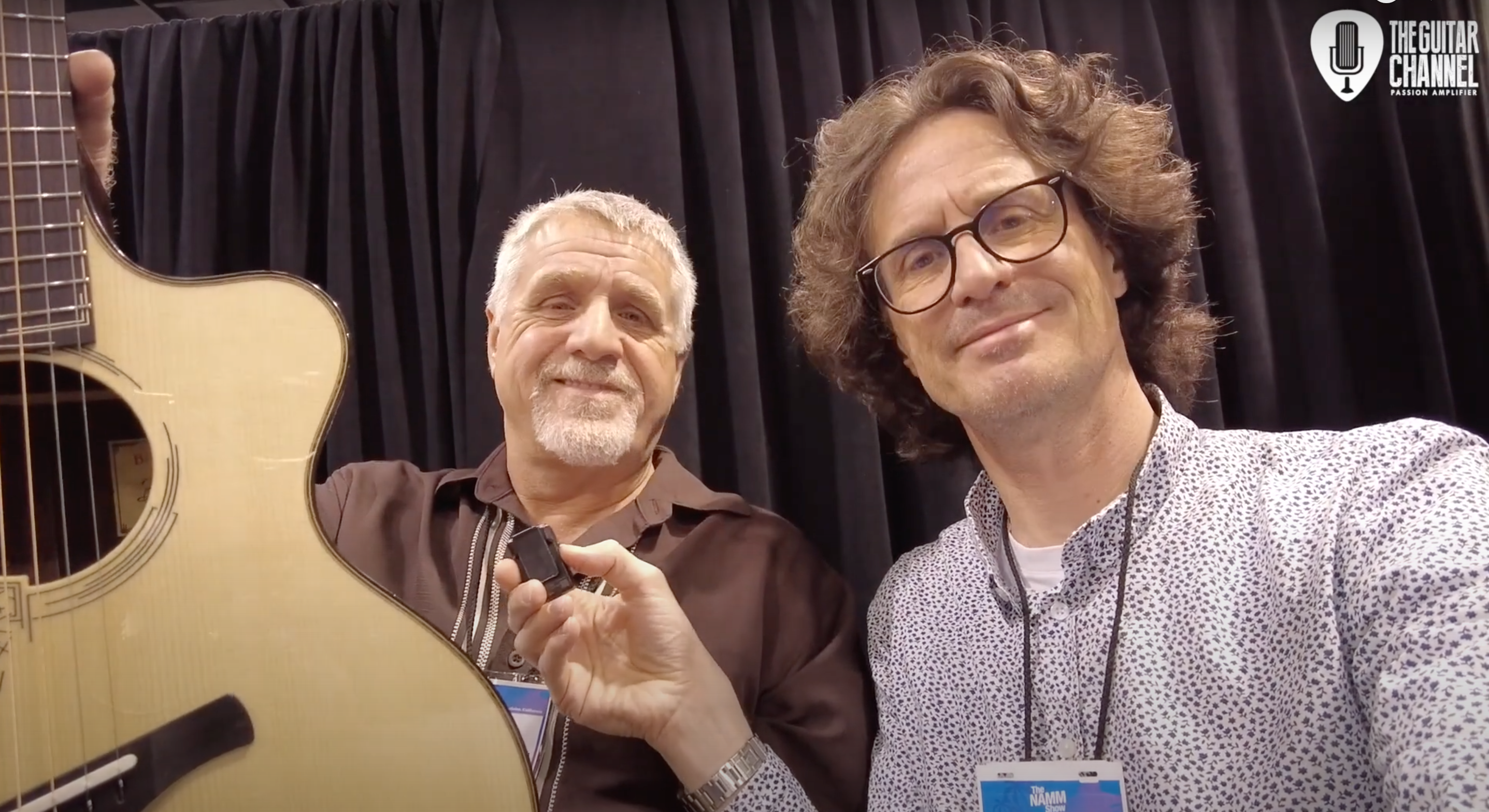This detailed image captures two men posing indoors against a black curtain backdrop, likely part of a podcast or radio setting. The man on the left, seemingly older with short gray hair and a goatee, holds up a light-colored wooden acoustic guitar with visible strings. He wears a brown collared shirt and a laminated name tag. The younger man on the right has brown curly hair, glasses, and dons a speckled long-sleeve jacket with a collar. He is holding something—possibly a clip or microphone—in his hand while also wearing a laminated pass. Both men are smiling slightly and looking down at the camera, suggesting the photo was taken from a lower angle. In the upper right corner, there is a logo and text that reads "The Guitar Channel: Passion Amplifier." The scene is filled with colors like tan, brown, black, light brown, white, and blue.